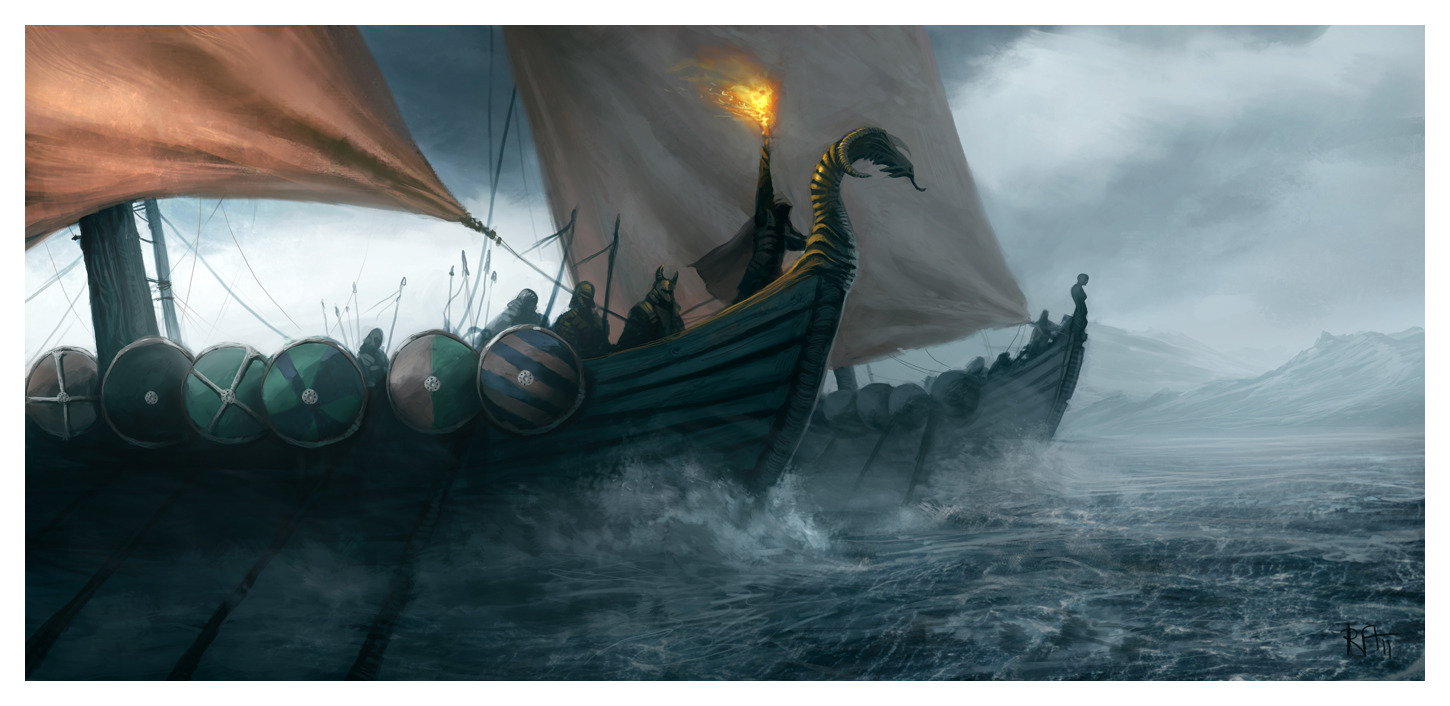This is a detailed painting of two Viking ships navigating through rough waters. The scene is dramatic, with turbulent waves crashing against the sides of these ancient longboats. In the foreground, one ship is prominently displayed with a dragon head at its prow and a beige sail partially visible. Warriors, recognizable by their Viking helmets, stand along the edges, their large round shields mounted on the sides of the ship, perhaps for protection. At the very front, a figure holds a burning torch high, possibly signalling to the shore or the other boat. The sky above is menacing with dark gray clouds, adding to the ominous atmosphere. In the background, another ship is seen with a white sail, but only partially visible. The entire scene is framed by distant, shadowy mountains, indicating that the ships are in a smaller body of water close to shore.